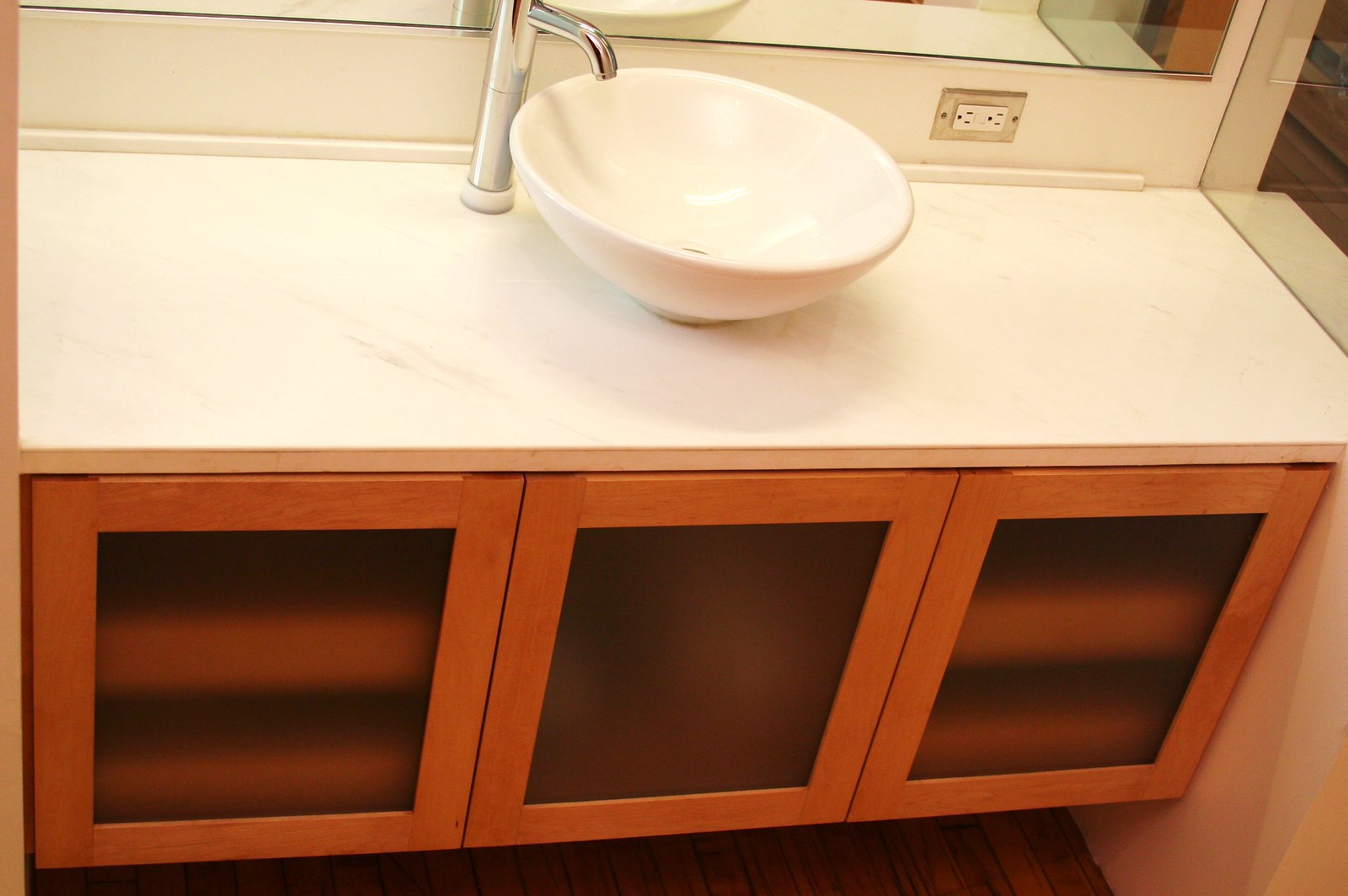This photograph showcases a contemporary bathroom design featuring a sleek and modern sink area. The sink rests atop an elegant white marble countertop that spans the width of the cabinetry below. The cabinetry consists of three doors framed in light wood, each with an inset of translucent glass. Behind the doors on the left and right are the fronts of two drawers, providing additional storage space.

To the left of the cabinetry, just the edge of the adjacent wall is visible, suggesting a confined yet cozy setting. On the right side, a large mirror extends from just above the countertop to the ceiling, creating an illusion of space and amplifying light within the room. An electrical outlet is positioned on the rear wall, which is similarly clad in the exquisite white marble, enhancing the cohesive aesthetic of the bathroom.

Sitting proudly atop the countertop is a stylish vessel sink, its bowl shape allowing the interior and exterior to be fully visible. Complementing this modern sink is a tall chrome faucet, adding a touch of elegance and functionality to the overall design. The seamless integration of these elements results in a visually appealing and highly functional space.